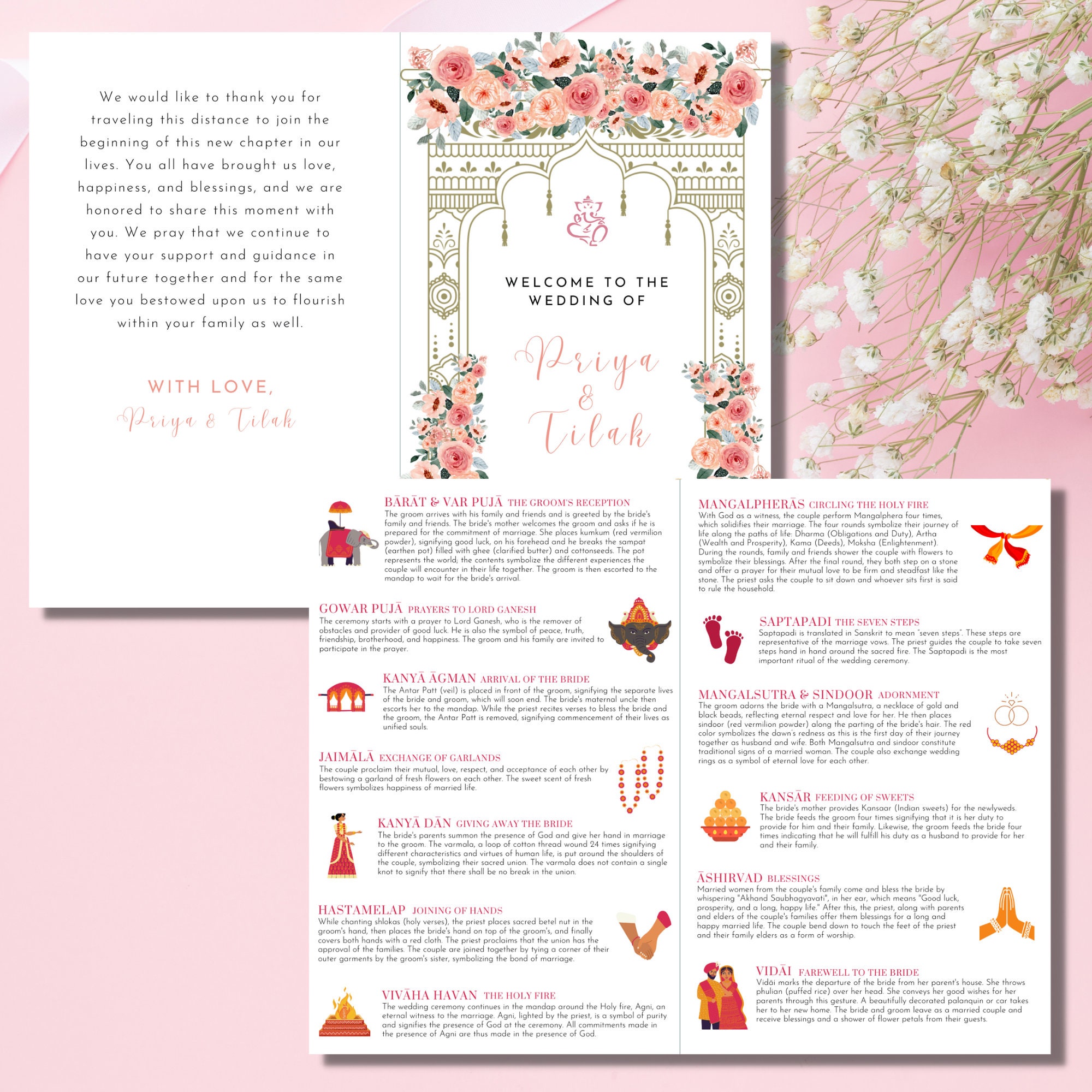The image features a stunning wedding invitation set against a soft pink background adorned with delicate pink flowers and green stems emerging from the top right corner. The invitation, elegantly opened, reveals a beautiful design reminiscent of a chapel's facade, framed by pretty pink flowers along the top and sides. 

In a graceful light orchid font, the text reads: "Welcome to the wedding of Priya and Tila." The heartfelt message continues, "We would like to thank you for traveling this distance to join the beginning of this new chapter in our lives. You all have brought us love, happiness, and blessings, and we are honored to share this moment with you. We pray that we continue to have your support and guidance in our future together, and for the same love you have bestowed upon us to flourish within your family as well. With love, Priya and Tila."

The inside of the invitation is equally detailed, featuring an array of small pictures and accompanying inscriptions, each one contributing to the rich tapestry of Priya and Tila's love story and the joyous occasion they are about to celebrate.